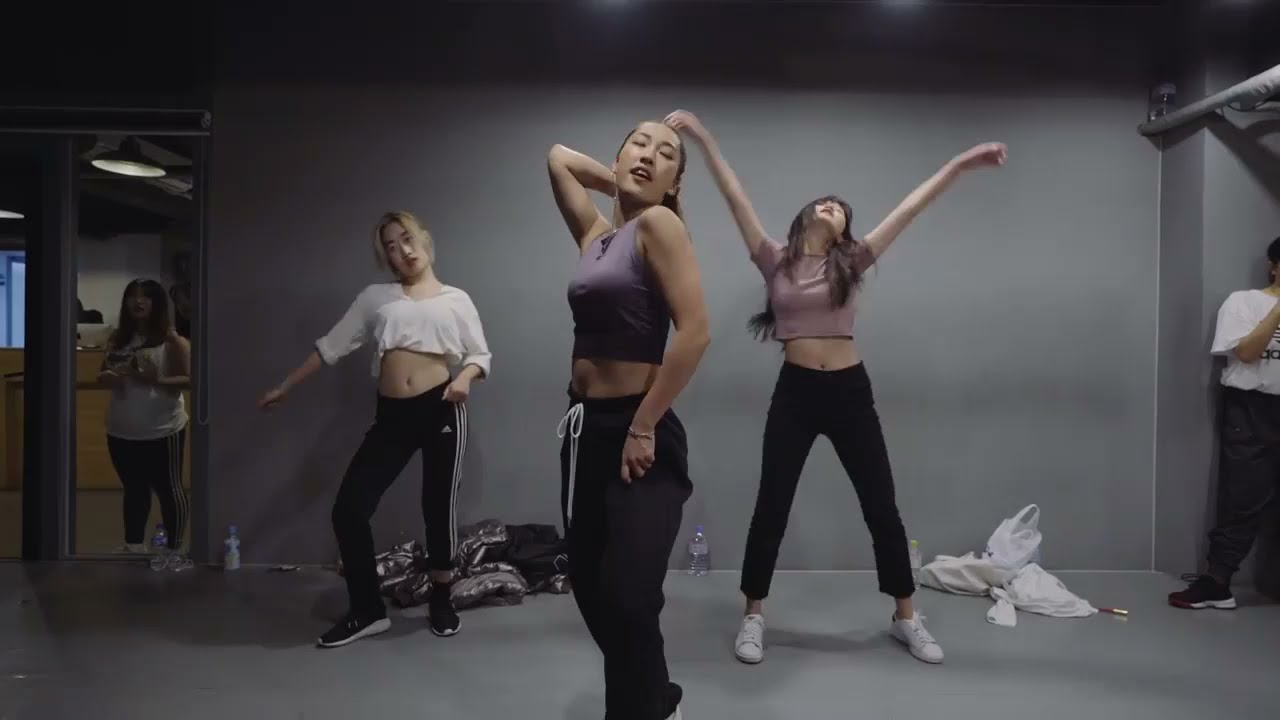The image depicts a vibrant scene inside a dance studio with a predominantly gray color scheme, characterized by its gray walls and floors. Centrally positioned are three women engaged in a dance routine. To the left of the middle stands a woman with medium-length blonde hair, dressed in a white crop top, black sweatpants, and black tennis shoes; she is poised mid-movement with her right arm extended to her side, her left arm bent, and her right foot up on her toes. Next to her, slightly turned left but facing forward, is another woman in a gray short top and black sweatpants with a white drawstring. She has her right arm bent behind her head and her left arm down beside her. To the right in the middle section of the image is a woman with long dark hair, a light-colored crop top, black sweatpants, and white tennis shoes. Her head is tilted back, looking upward with both arms raised and extended outward. 

On the right edge of the image, a person is partially visible, wearing a white t-shirt, black pants, and black shoes. To the far left, just behind the central women, a mirror on the wall reflects another woman with a white top, black pants, and shoulder-length dark hair. The studio floor behind the central figures is scattered with bags, possibly backpacks or duffel bags, along with several bottles arranged against the back wall, hinting at a lively session. The scene suggests a bustling dance class or practice session, filled with dynamic movements and a sense of organized chaos.